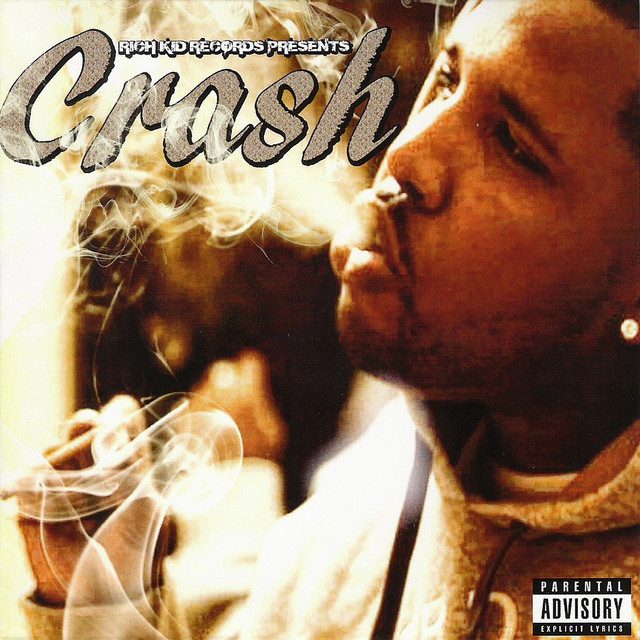The image is an album cover for a hip-hop artist, featuring a black individual blowing smoke from a marijuana blunt or cigar held in his right hand. The man, who has a beard and a stud earring, is wearing a gray shirt or hoodie. The cover has a noticeable presence of smoke circulating throughout the left-hand side of the image. In the upper left corner, in small white text, it reads "Rich Kid Records Presents." Directly beneath that, the title "CRASH" is displayed in a prominent silver-gray or cursive-stylized font. The bottom right corner features a parental advisory warning for explicit lyrics. The overall color scheme consists of various shades of brown and tan, contributing to a cohesive and atmospheric look.